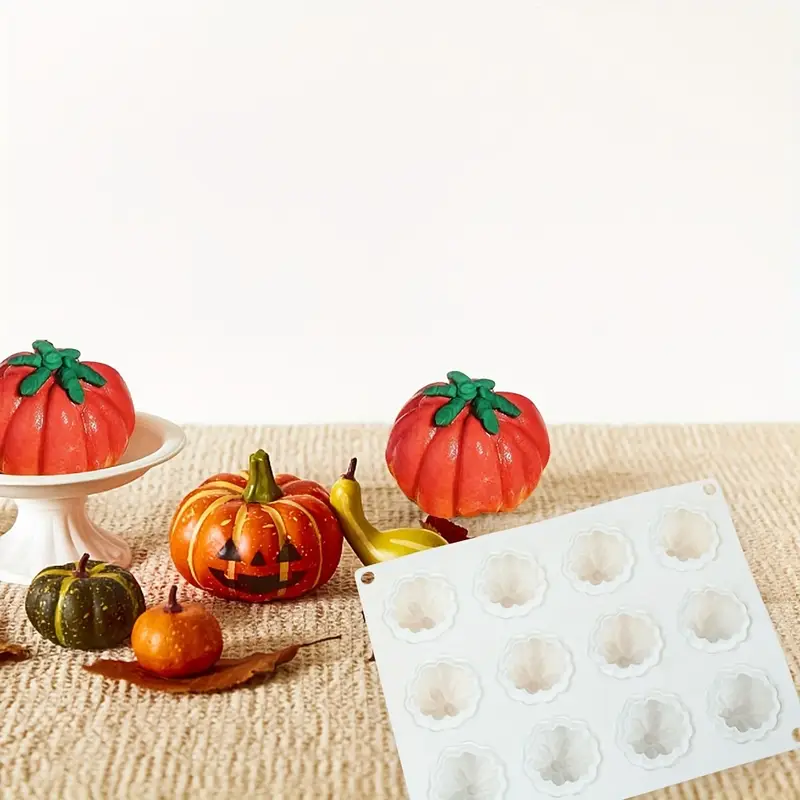The photograph features an autumn-themed place setting on a woven beige tablecloth that occupies the lower half of the frame, with a stark white wall in the background. Centralized on the left is a white dish cradling a reddish-orange gourd. Adjacent to this, towards the table's center, sits an orange plastic pumpkin embellished with a black jack-o'-lantern face. To the left and slightly lower, a dark green and light green gourd adds a pop of cooler color. Moving to the right, an orange fruit, possibly a tomato, rests atop a crispy brown leaf, adding to the fall aesthetic. Leaning against the jack-o’-lantern is a lime green and olive-green striped gourd with a slender neck. Above this, a yellowish-orange gourd with green leaves adds variety. In the bottom right quadrant, a white mold tray designed to shape twelve small pumpkin-like forms, each with scalloped edges, is placed. Scattered autumn leaves further enhance the festive Halloween scene.